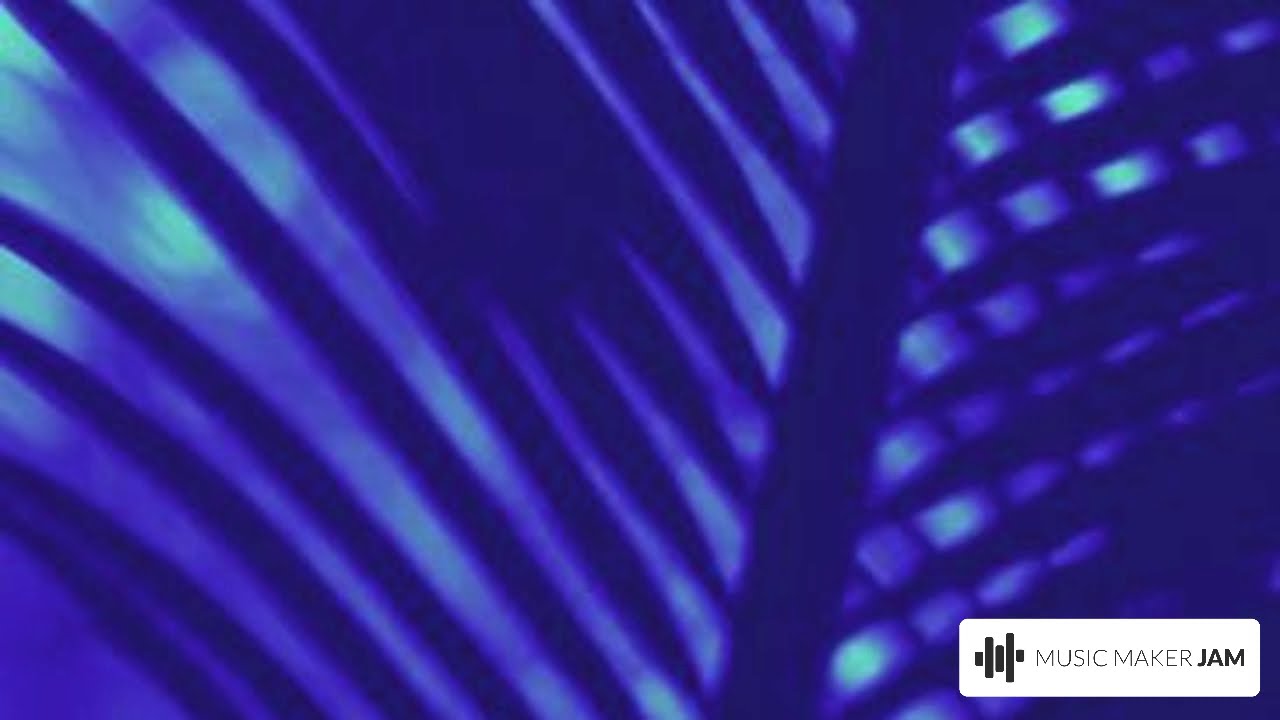The image features a navy blue, leaf-like pattern, reminiscent of a palm branch. This pattern consists of a central stem with diagonal veins or smaller stems extending towards the left and right, creating a textured effect that spans across a predominantly blue background. In the background, there's a gradient of lighter blue and turquoise hues, giving the impression of light glowing through the leaf structure.

In the lower right-hand corner of the image, there's a white rectangle containing the text "MUSIC MAKER JAM." The words "MUSIC MAKER" are in a light font, while "JAM" is bolded, all in uppercase sans-serif letters. To the left of the text, there are vertical black bars that resemble audio equalizer levels, symbolizing sound waves. The overall aesthetic of the image suggests it may be designed as a computer wallpaper or an advertisement for an audio-related service, emphasizing a blend of natural and digital elements.